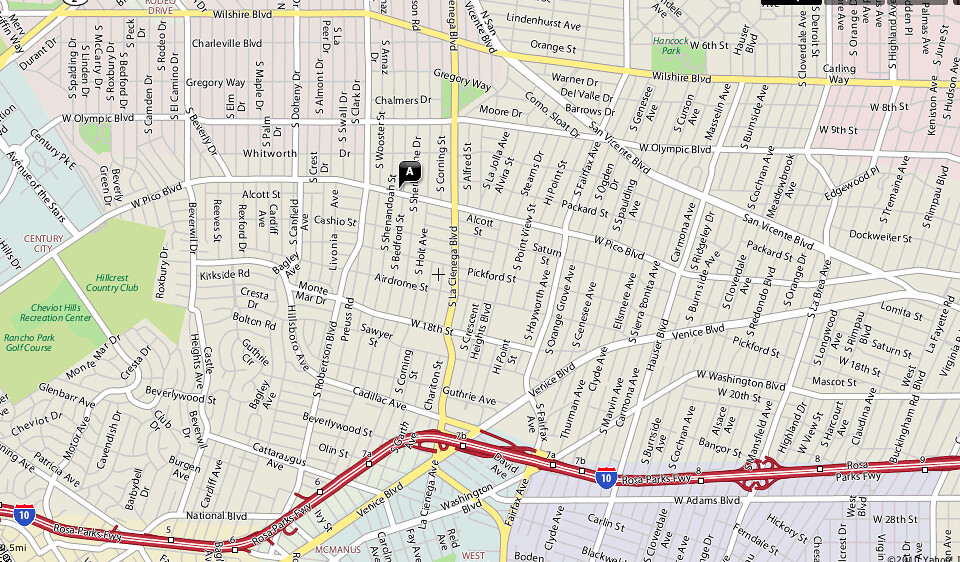This image showcases a detailed map focusing on a specific area of a city. Centrally, there is a distinct black bubble with the letter "A" pointing down at a location on South Shenandoah Street, suggesting a notable or destination point. Prominent roads are highlighted: Wilshire Boulevard, marked in yellow, runs horizontally and intersects with South La Cienega Boulevard, also in yellow, indicating busy streets. Towards the bottom, the map features the Rosa Parks Freeway in a bold red strip, signifying a major highway.

Scattered across the map are several key landmarks and recreational sites. Olympic Boulevard is near a visible park, while Hancock Park stands out prominently. The Hillcrest Country Club, a recreation center, and the Rancho Park Golf Course are also clearly marked, emphasizing the area's mix of residential zones and recreational facilities. The map provides a comprehensive view of the neighborhood, with both bustling streets and serene green spaces.